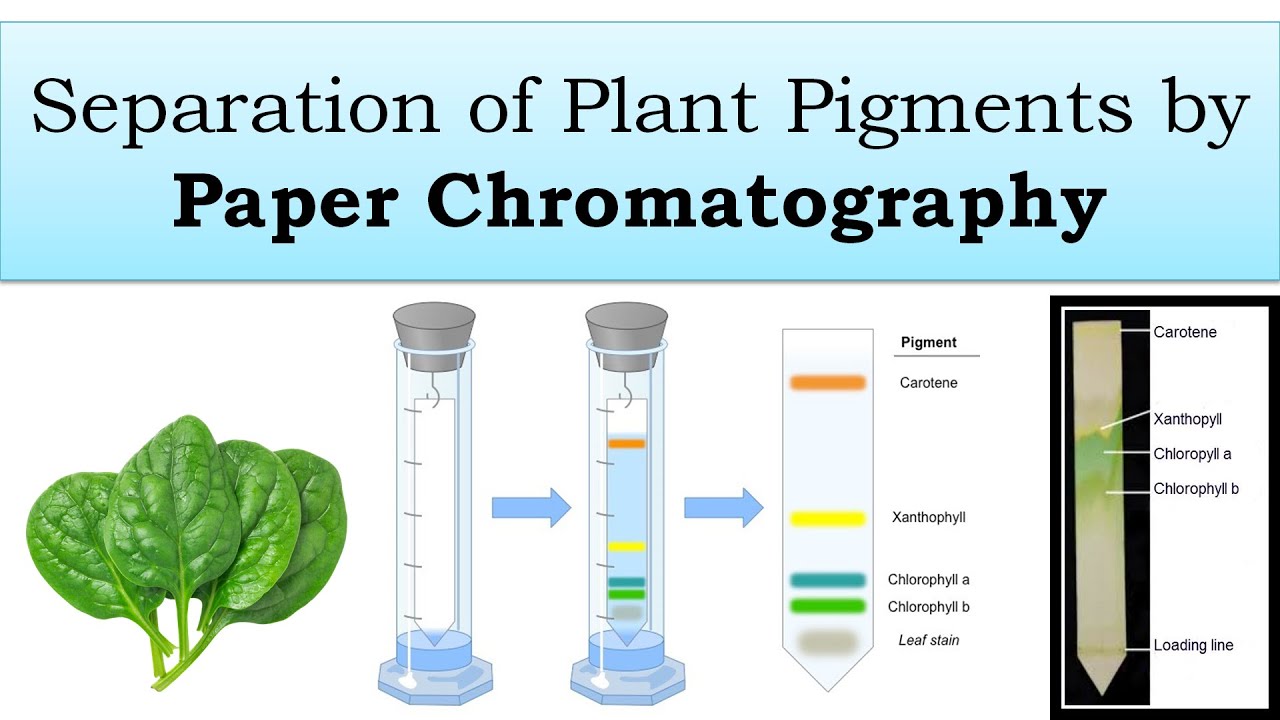The infographic titled "Separation of Plant Pigments by Paper Chromatography" is set on a blue background. At the top, the bold text emphasizes the process name. On the left side of the image, four vividly green spinach leaves are arranged in a fan. Next to the leaves, there are two test tubes (or vials). An arrow points from the first vial, which contains a long white strip of paper, to the second vial, where the paper strip has undergone a dyeing process. This paper now shows distinct colored bands representing various pigments. In the middle, the labeled colored bands are as follows: a red stripe for carotene, yellow for xanthophyll, blue for chlorophyll A, green for chlorophyll B, and a gray stripe for leaf stains. On the far right, a closer view of the dyed strip showcases these pigments clearly, accompanied by a more realistic photograph of the same colored bands, further illustrating the separation of plant pigments.